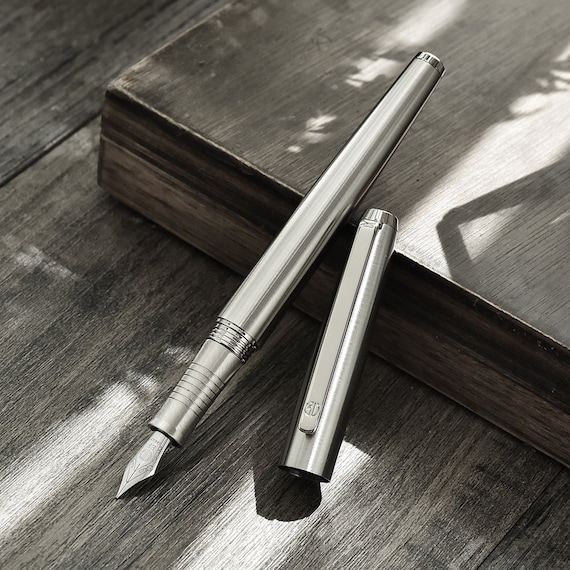The black and white photograph depicts an elegant, silver-colored fountain pen with a sharp tip placed diagonally from the top right to the bottom left of the image. The pen, which is open and shows the nib at the bottom, rests against a small piece of wooden block atop a textured wooden tabletop. The polished and minimalist design of the pen contrasts with the natural variations in the wood. Sunlight streams in from the side, casting distinct shadows and creating the silhouette of flowers against the wooden background, accentuating the outdoor setting of the scene.